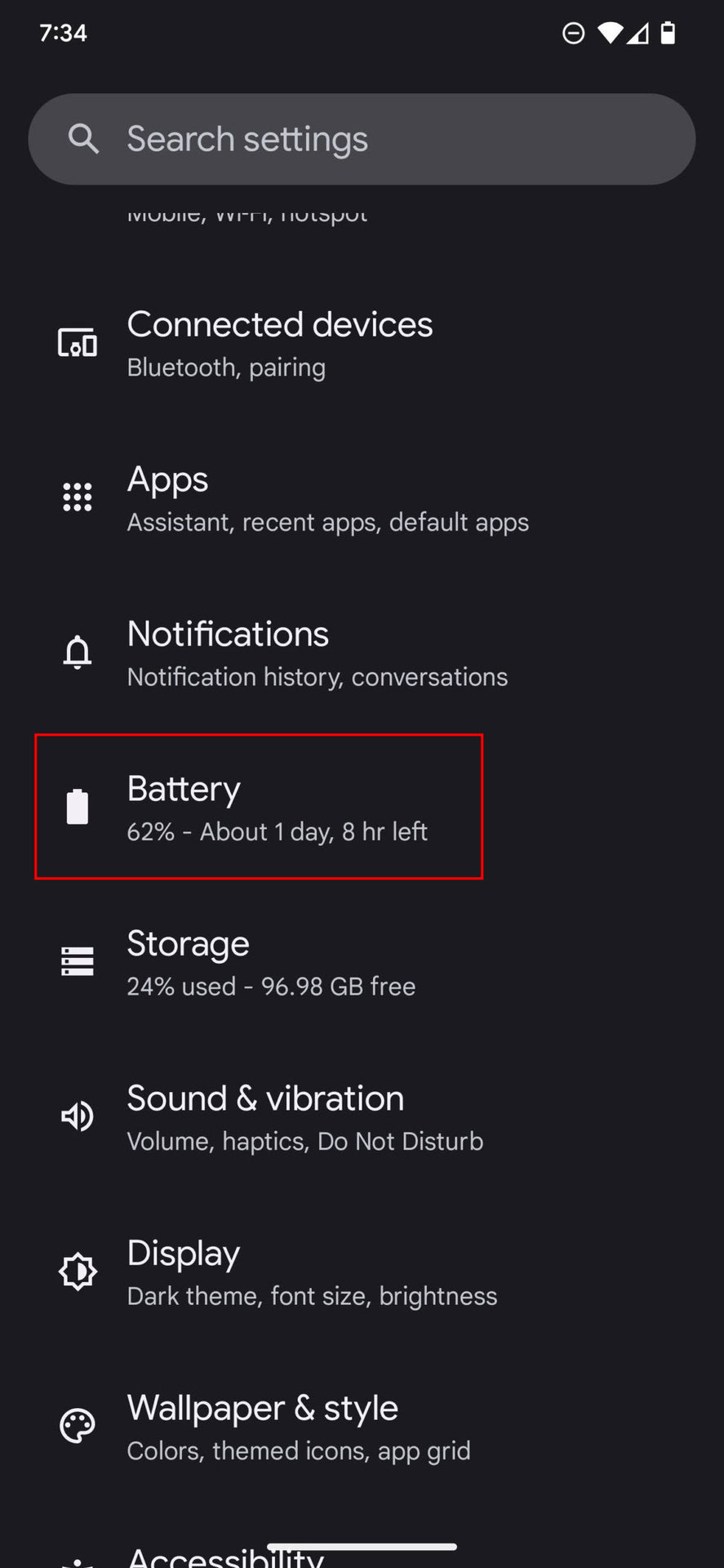The screenshot displays a cell phone's settings menu against a black background with white text. At the top left corner, the time reads "7:34," while the top right corner shows several icons: the Do Not Disturb icon (a circle with a horizontal line), the Wi-Fi icon, signal reception bars, and the battery icon. Below these, there is a gray search bar adorned with a magnifying glass icon and the words "Search settings" in white.

Just below the search bar, the lower half of the text "Mobile Wi-Fi hotspot" is visible. This is followed by a list of nine menu options, each written in white text accompanied by a corresponding icon. The options, in order, are:
1. Connected devices
2. Bluetooth pairing
3. Apps
4. Assistant
5. Recent apps
6. Default apps
7. Notifications
8. Notification history conversations
9. Battery (highlighted with a red rectangle), showing "62%, about one day eight hours left"

Following the battery option, additional menu items are visible:
10. Storage, displaying "24% used, 96.98 GB free"
11. Sound and vibration, listing "Volume, haptics, do not disturb"
12. Display, mentioning "Dark theme, font size, brightness"
13. Wallpaper and style, listing "Colors, themed icons, app grid"

The battery option is specifically emphasized with a red outline, indicating it is currently selected.